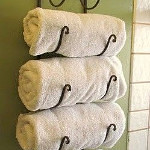The image is a small, square photograph showcasing three white towels rolled up in a cylindrical shape and stacked vertically on a hanging black metal towel rack. Each towel is securely held in place by its own set of metal hooks, which arc around the bottom and form outward-facing loops at the ends. The rack is mounted on a light green wall, and to the right, there is a partial strip of white tile that descends vertically. The close-up shot cuts off the top and bottom of the rack, making the exact structure of the upper loops unclear.